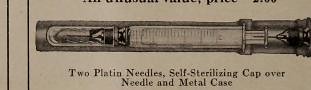The image appears to be a close-up of a black-and-white illustration of a hypodermic needle, possibly taken from a dated and yellowing magazine or catalog. The needle, oriented horizontally and pointing to the left, is enclosed by a self-sterilizing cap. The central positioning of the needle highlights its design, including a small reservoir for liquids. Below the needle, the text reads: "Two platen needles, self-sterilizing cap over needle and metal case," with the last sentence placed on a second line. Above the needle, partially obscured text suggests additional context or instructions, consisting of five incomplete words. The background of the image is a light brown, contributing to the aged appearance of the page.